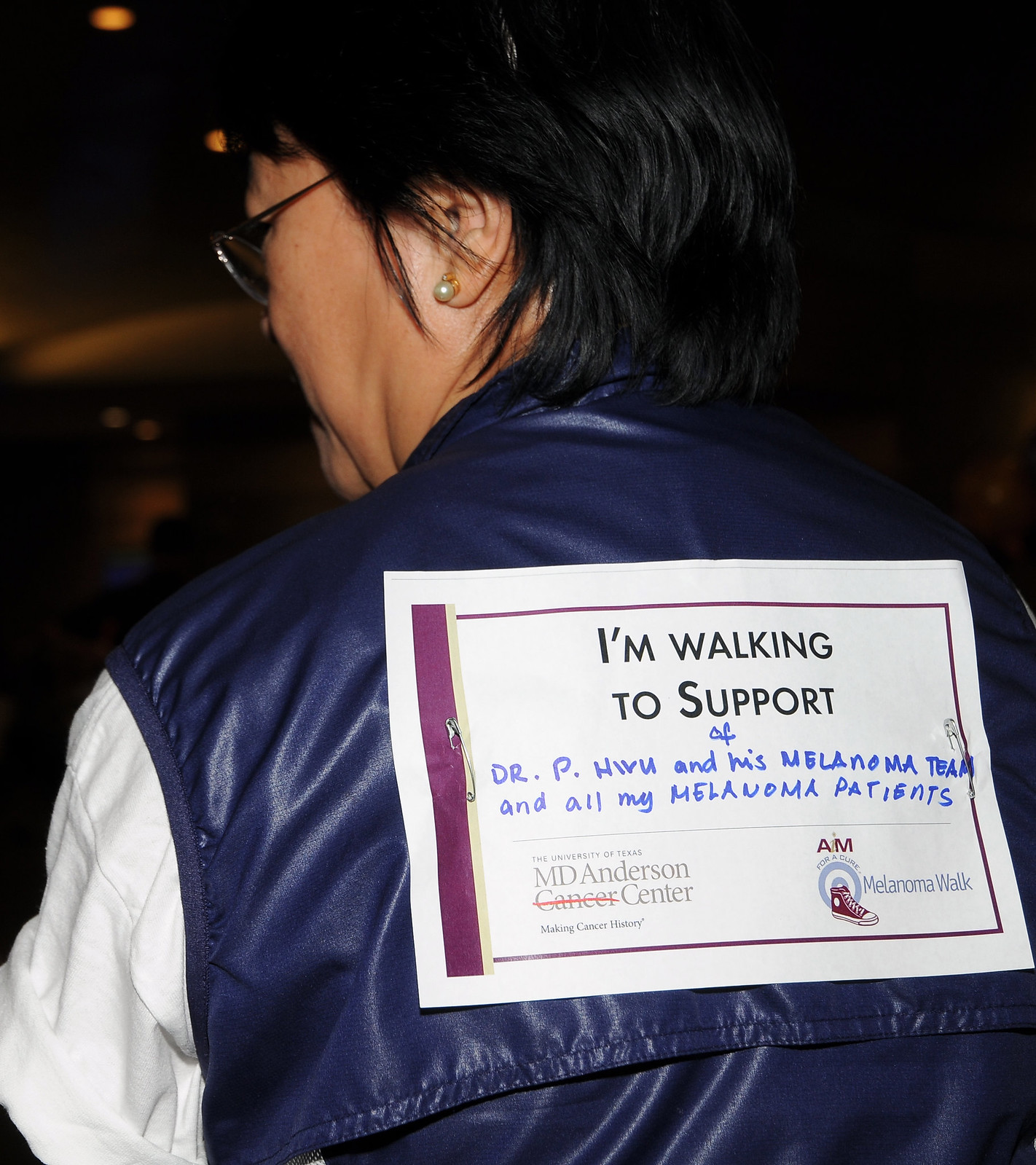This nighttime photograph captures a close-up of a woman, predominantly visible from the shoulders up. She stands in the very center of the image, facing away from the camera, slightly turning her head to the left. The woman, who appears to be middle-aged and Asian, is characterized by her short black hair, pearl earring in her left ear, and glasses. She's donning a leather-type jacket predominantly blue with white sleeves. Safety pins attach a piece of paper with a purple border to her jacket. The paper bears a printed message in black text: "I'm walking to support," followed by a handwritten note in blue marker: "Dr. P. Hiru and his melanoma team and all my melanoma patients." The MD Anderson Cancer Center logo is featured in the lower left, while a shoe icon and the words "Melanoma Walk" are present in the bottom right. This suggests she participates in the University of Texas MD Anderson Center's Aim for a Cure Melanoma Walk, helping to raise funds and awareness for melanoma research and treatment.